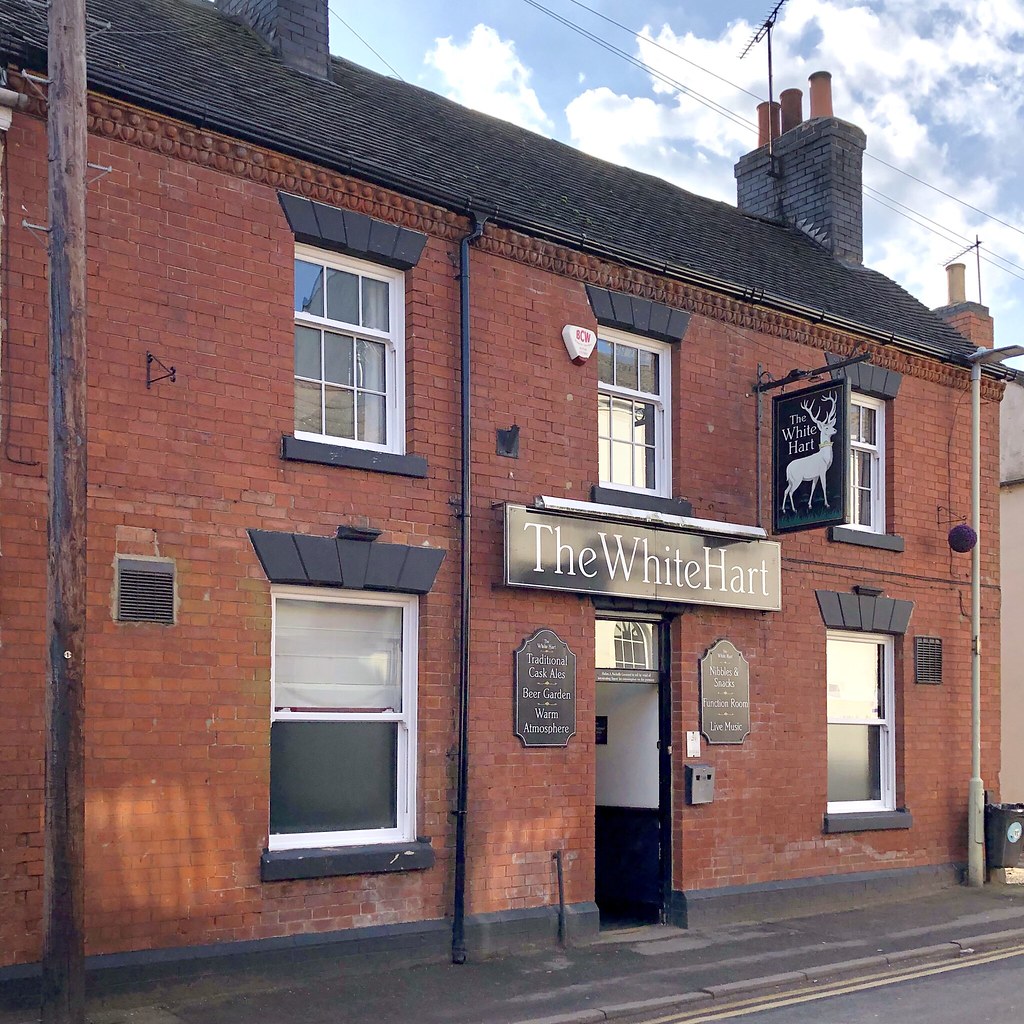The image captures the exterior of an old-fashioned, two-story brick building, likely a pub in the UK, known as "The White Heart." The orangish-red brick structure boasts a roof with black tiles and a chimney featuring three spouts. The building presents white-framed windows, three on the upper floor and two on the lower floor, flanking an open doorway. Above the doorway hangs a wooden sign that reads "The White Heart" in white letters. On either side of the entrance are two menu boards listing offerings such as traditional cask ales, a beer garden, nibbles and snacks, a function room, live music, and a warm atmosphere. A side banner extends from the building, depicting a white deer, or elk, against a black background, standing on green grass. The narrow sidewalk in front is a dark gray, leading to the narrow street visible in the image. Above, the blue sky filled with clouds mirrors the quaint charm of the historic establishment. Telephone poles can be seen in the background, adding to the rustic ambiance.